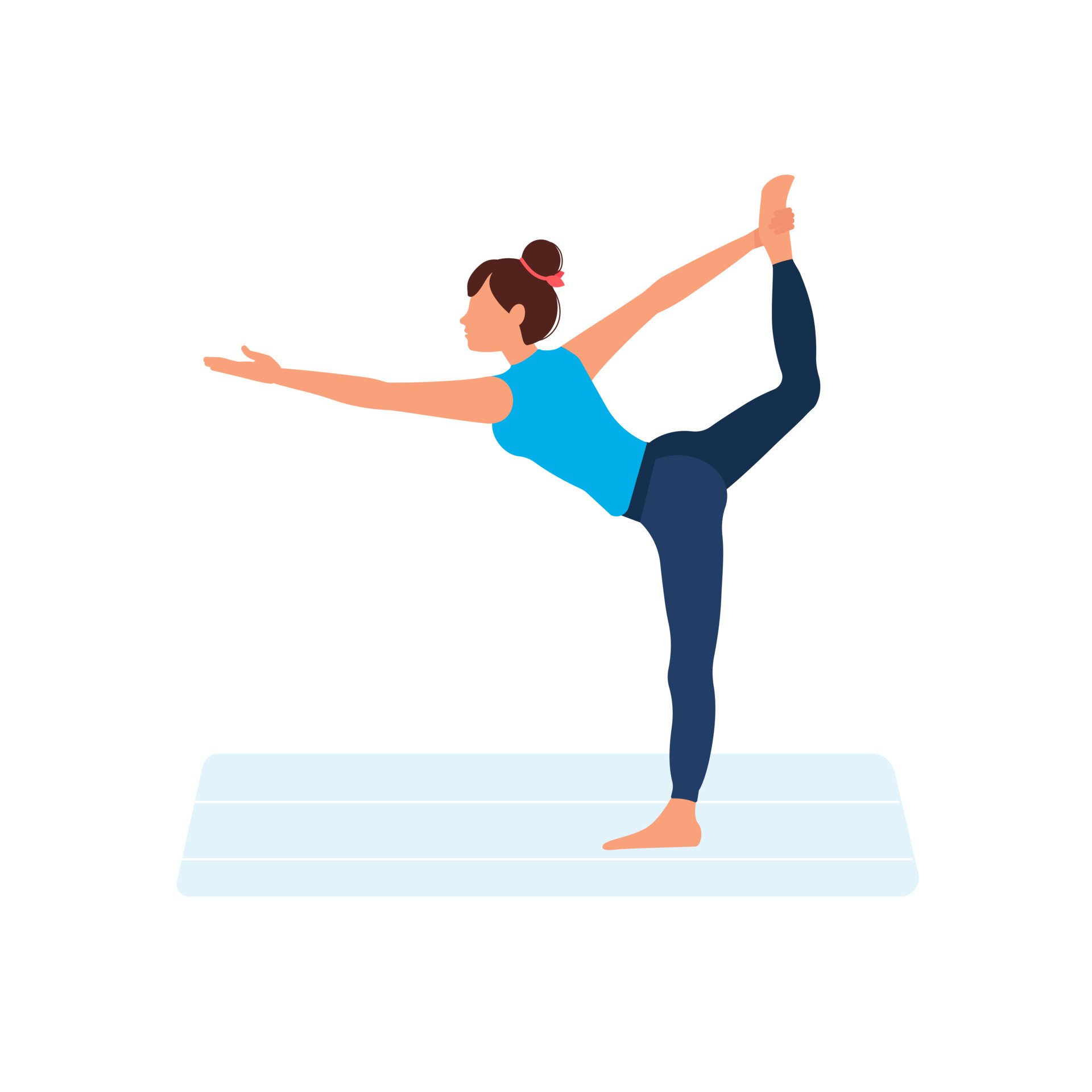The image is a color illustration in portrait orientation, depicting a woman performing an advanced yoga pose on a very pale blue yoga mat. The woman, facing left, is balancing on her straight left leg while her right leg is bent backward, and she holds her right foot with her right hand. Her left arm extends forward, enhancing her lean-forward posture. The illustration features a white background, emphasizing the simplicity and focus on the figure. She has dark brown hair tied in a bun secured with a red ribbon at the base. Her outfit consists of a robin's egg blue tank top that meets the top of her navy blue yoga pants, which appear darker on the right leg. The woman’s skin has a dark peach hue and lacks facial features, giving the image a minimalistic and stylized feel.